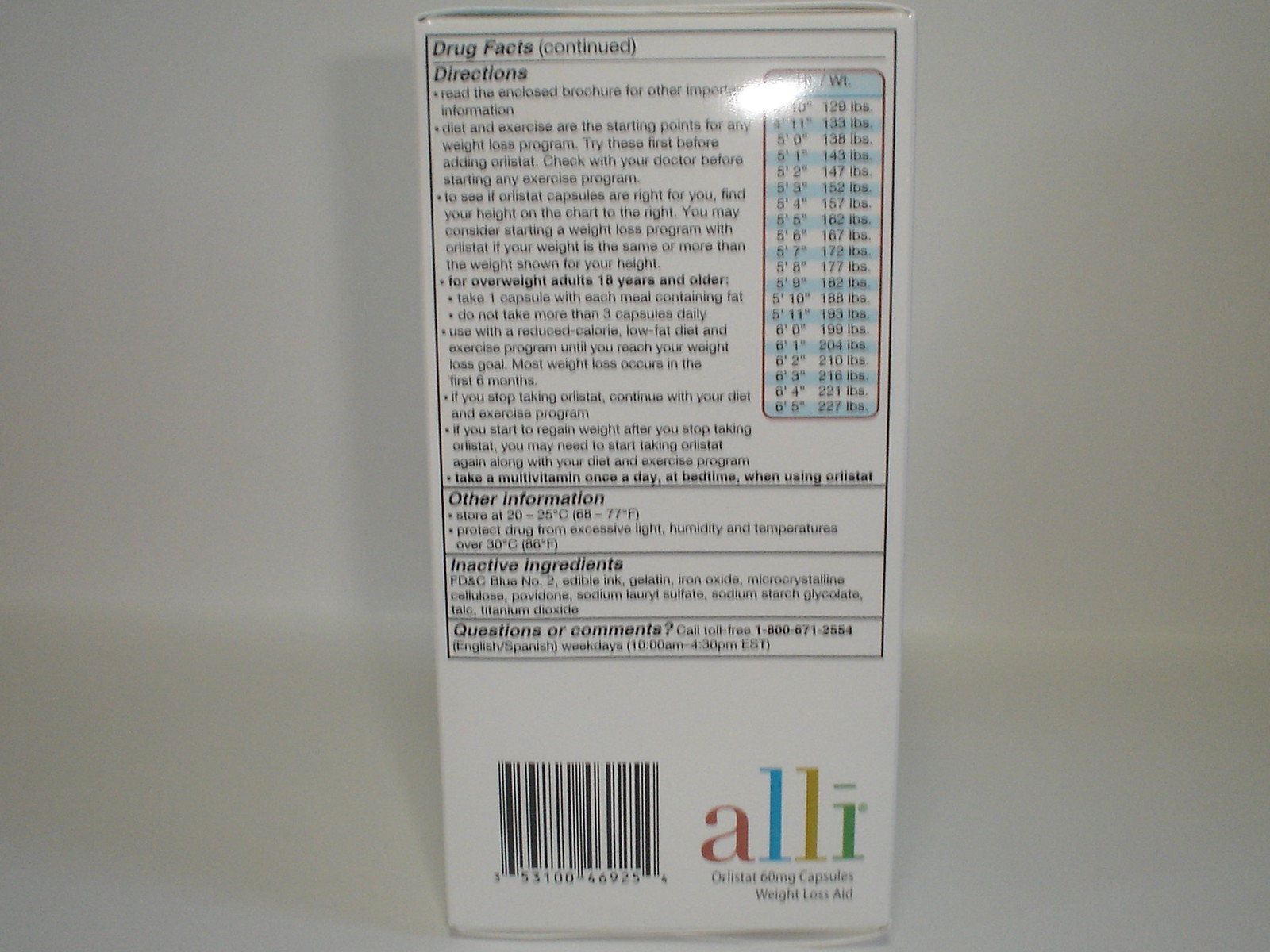A high-resolution photograph features a box of medication prominently displayed against a pristine white surface. The box, primarily white with black text, is designed with a rectangular blue, white, and black height and weight chart on the front. A barcode is visible at the bottom of the front side, accompanied by colorful letters: a red 'A', a blue 'L', a gold 'L', and a green 'I'. The box is labeled "60 mg Capsules" in clear black font, indicating it is a weight loss aid. The reverse side of the box is densely packed with instructions and drug facts in black font, providing comprehensive directions. The weight chart on the back delineates ranges from approximately 120 pounds to 227 pounds, catering to various weights for dosage guidance.